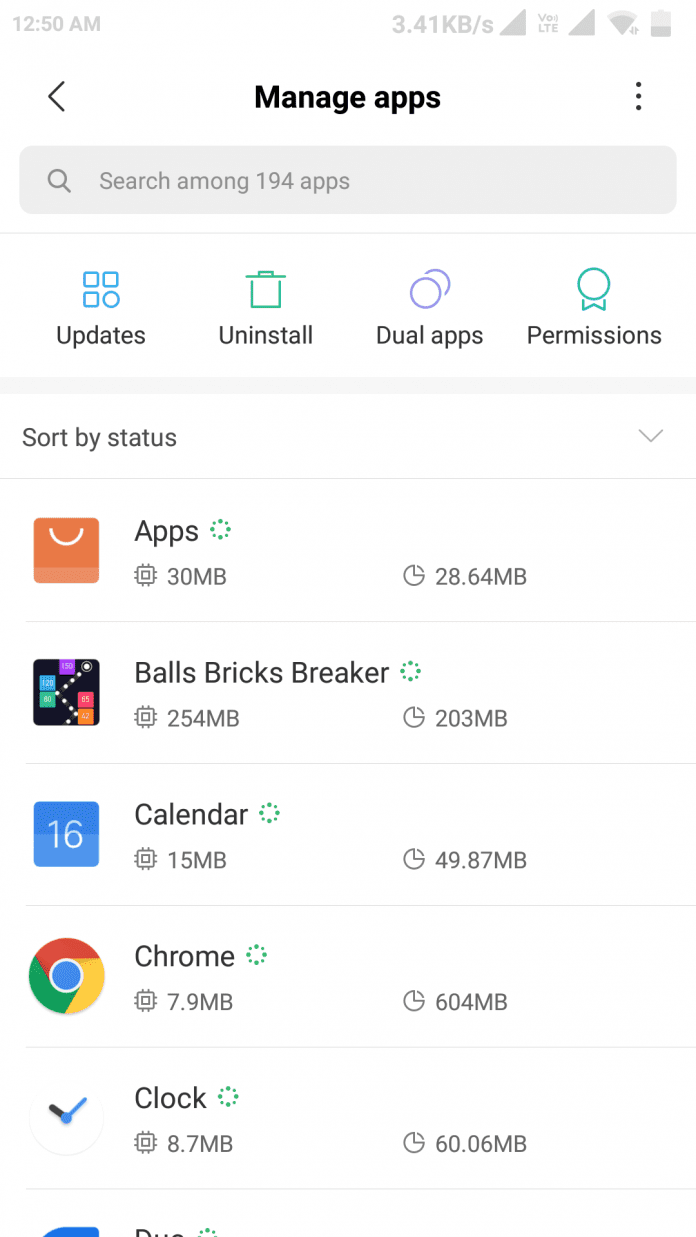This image depicts a screenshot taken from a smartphone, displayed against a white background. At the very top of the image, a grey status bar shows the time "12:50 AM," along with "3.41 KB" and a symbol resembling a forward slash or 'S'. Below the status bar, in bold black letters, it reads "Manage Apps." Beneath this title is a search bar that prompts, "Search Among 194 Apps."

Following the search bar are four icon buttons labeled "Updates," "Uninstall," "Dual apps," and "Permissions," each represented by distinctive icons. "Updates" is shown with a square grid pattern, "Uninstall" is depicted by a trash can, "Dual apps" features overlapping circles, and "Permissions" is indicated by a circled banner resembling a medal.

Further down, a section titled "Sort by status" appears. On the left side of this section, various app icons are listed along with their names. Some of the entries include:

- "31 MB" and "28.64 MB"
- "Balls Bricks Breaker" with sizes "254 MB" and "203 MB"
- "Calendar" with "15 MB" and "49.87 MB"
- "Chrome" with "7.9 MB" and "604 MB"
- "Clock" with "8.7 MB" and "60.06 MB"

Each of these items appears to detail the storage usage of the respective applications, indicated in megabytes (MB).